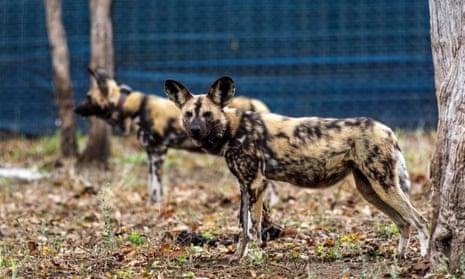In this photograph, two African wild hunting dogs stand on the ground within a blue fenced enclosure, possibly a zoo. The animals, often confused with hyenas, display a distinct coat pattern with brown and black markings, black spots, and lines. The closest dog to the viewer faces left, but its perked ears and gaze are directed towards the camera, revealing a black face with a stripe down its forehead. The other dog stands slightly behind, facing left and providing a clear side view. The ground they stand on is mostly barren soil mixed with dry leaves, patches of green and yellow weeds, and dandelions. The area features a couple of tree trunks observable to the left and the right, with some leaves likely having fallen from these trees. In the background, the blue, cross-hatched fence completes the scene, indicating an enclosed space.